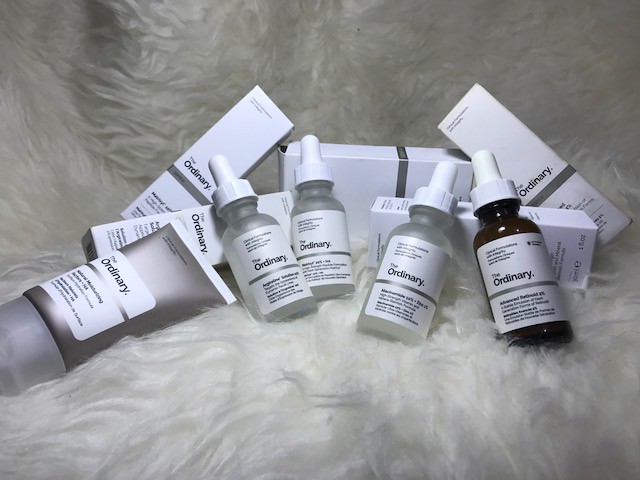This landscape-oriented photograph meticulously showcases skincare serums from the brand "The Ordinary." Set against a luxurious, fluffy Greek flokati background, the image exudes a sense of opulence and comfort. The flokati blanket is artfully draped against what appears to be a counter or display stand, extending upwards to form a plush backdrop. Central to the arrangement are four glass vials equipped with medicine droppers alongside a sleek plastic tube, each product distinctly labeled with "The Ordinary." The vials are adorned in shades of gray and dark brown, while the tube shines in a metallic silver hue. Carefully positioned behind the products are their respective boxes, creating a small, neat tower that adds to the visual appeal and emphasizes the brand's aesthetic. This is a thoughtfully arranged display, clearly intended for promotional purposes rather than an everyday medicine cabinet. Each product likely offers unique benefits for skincare, targeting areas such as the eyes and skin.